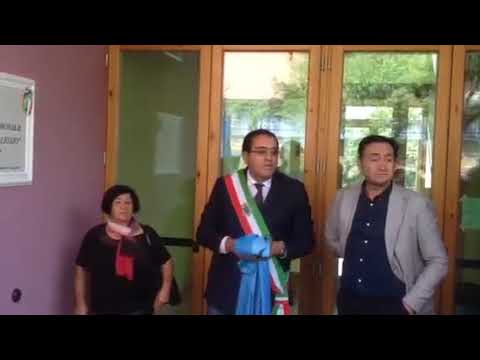This horizontally aligned rectangular photograph, bordered with thick black strips on the top and bottom, showcases three individuals standing in front of a double door entry with wooden frames and glass panes. The backdrop features a pink wall on the left with an indiscernible white-framed picture.

From left to right: the first person is a short woman with black hair that slightly passes her ears. She is dressed in a black short-sleeved shirt and accessorized with a distinctive multi-colored scarf in pink, black, and red tied around her neck. She appears to be holding a purse. The middle individual is a tall man in his early 40s, wearing glasses and a dark suit—likely black or navy blue—with a matching tie. Draped diagonally across his torso is a vibrant sash of red, white, and green, reminiscent of a country's national colors, possibly Mexico. He also clutches a blue ribbon in his hand. To the right, another man stands, dressed in a beige sport coat over a navy blue collared shirt with white buttons. All three individuals are gazing slightly to the right, and in the reflection of the glass doors behind them, a glimpse of trees outside is visible.